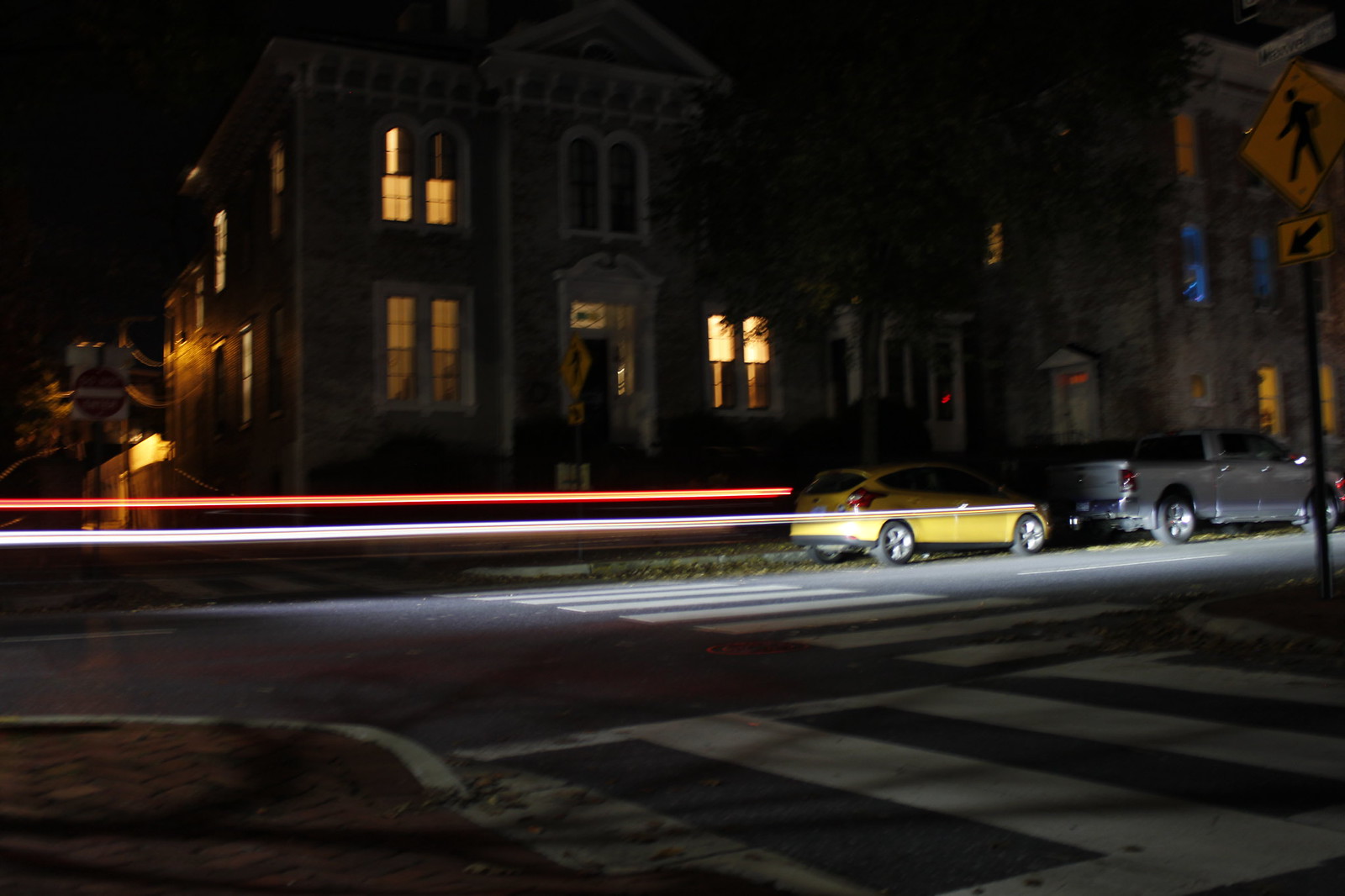A nighttime photograph captures a large house situated on a main road. The residence is fronted by two separate sidewalks, one directly opposite and one immediately in front. Parked in front of the house are two cars, one yellow and the other grey. The image appears digitally edited, featuring two distinct beams of light emanating from the yellow car—one white and projecting forward, the other orange and radiating to the background. Despite most interior lights being dimmed, a few yellow lights are visible through the windows, casting a subdued glow. The foreground of the image shows patches of grass interspersed with dust and scattered leaves, adding texture to the scene.